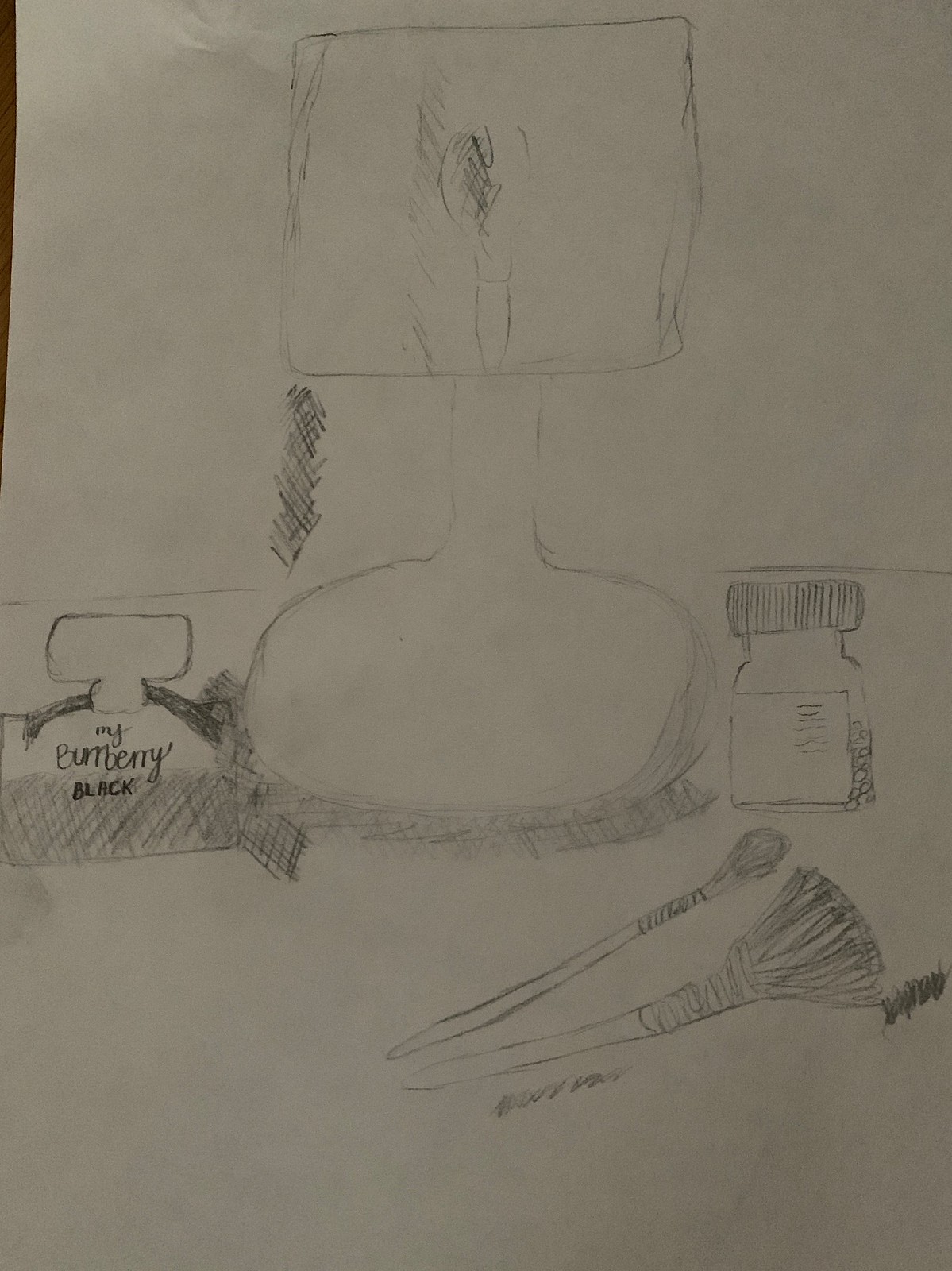This intricate pencil sketch, delicately rendered on white paper, portrays a collection of items typically found on a vanity table. Central to the composition is a small lamp, which features a round base, a slender neck, and a distinctive square lampshade. To the left of the lamp stands a bottle of cologne, characterized by its thick stopper top and semi-circular shape. The label on the bottle clearly reads "My Burberry Black." Opposite the cologne bottle is another container, possibly a medicine bottle, identifiable by its ribbed plastic lid. In the foreground, two makeup brushes are prominently displayed: one is a voluminous brush with a thick handle, and the other is a much smaller, slender brush. Each element in the sketch is meticulously detailed, capturing both the form and texture of the vanity table items.